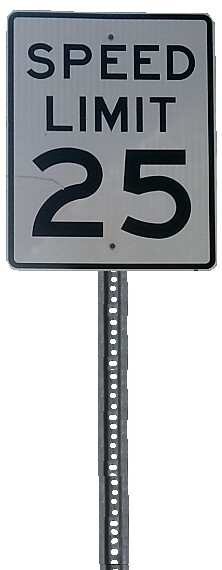This photograph features a standard rectangular speed limit sign set against a white background. The sign itself, though typically white, appears in a light gray shade likely due to lighting or reproduction effects. Encircled by a narrow black border, the sign is vertically oriented and has the text "SPEED" on the first line and "LIMIT" on the second line, both in capital letters. Below the text, the speed limit of "25" is displayed in much larger characters. Two small, circular bolts are visible at the top corners, securing the sign to a perforated metal post. The post, designed with multiple holes to allow versatile attachment options, anchors the sign firmly in place.